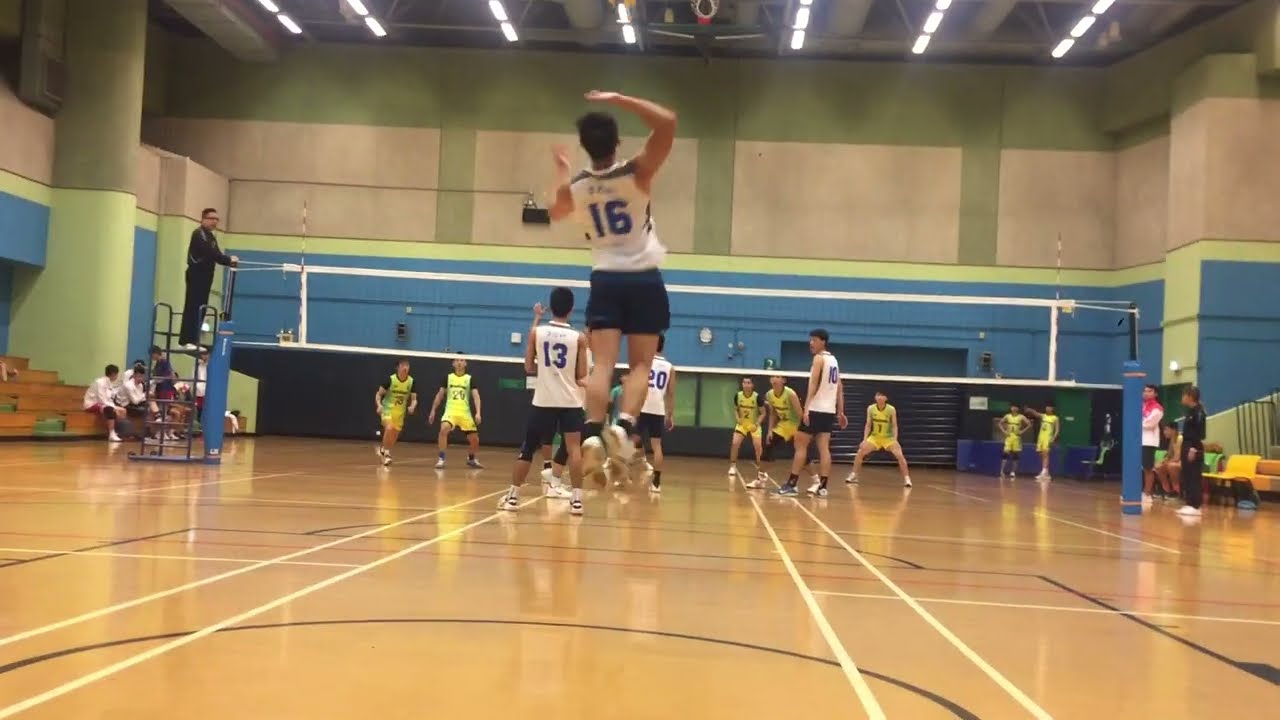The image captures an indoor volleyball game set in a gymnasium with a tan, shiny wooden court marked by red, white, and black lines. Approximately 10 young male athletes, possibly high school students aged 16 to 20, are engaged in the game, with one team dressed in white jerseys featuring blue lettering and black shorts, while the other team wears greenish-yellow jerseys. Positioned prominently in the center is a volleyball net, where a referee dressed entirely in black stands on a ladder with a whistle in his mouth, overseeing the game. The gym is enveloped by a blue-and-pale-green wall with tan and darker green sections, and features sideline bleachers where spectators and coaches can be seen. The overall scene is energetic and athletic, highlighting a competitive match in progress.